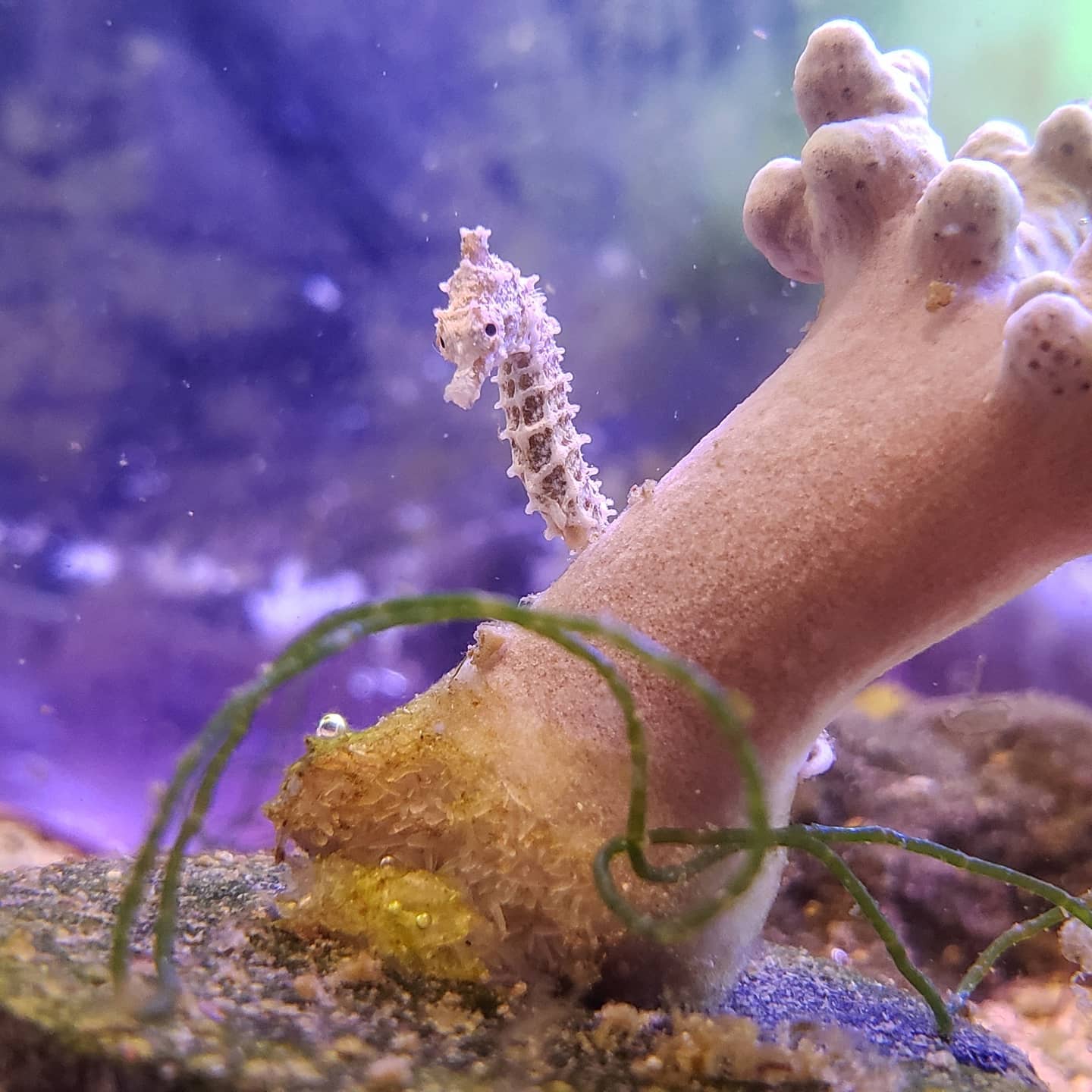The image is a high-quality, zoomed-in photograph depicting a mostly white seahorse with some pinkish tan hues, peeking out from behind a coral structure. The coral is pinkish and is situated in the mid-ground, while some green sea vegetation is seen in the foreground. The background is a dark purple-blue with white specks floating in the water, hinting at an underwater setting. The scene appears to be set in an aquarium or possibly in natural waters, with the light coming from the top right, casting a gentle glow onto the seahorse. The blurred background emphasizes the seahorse, making it the clear focal point of the image.